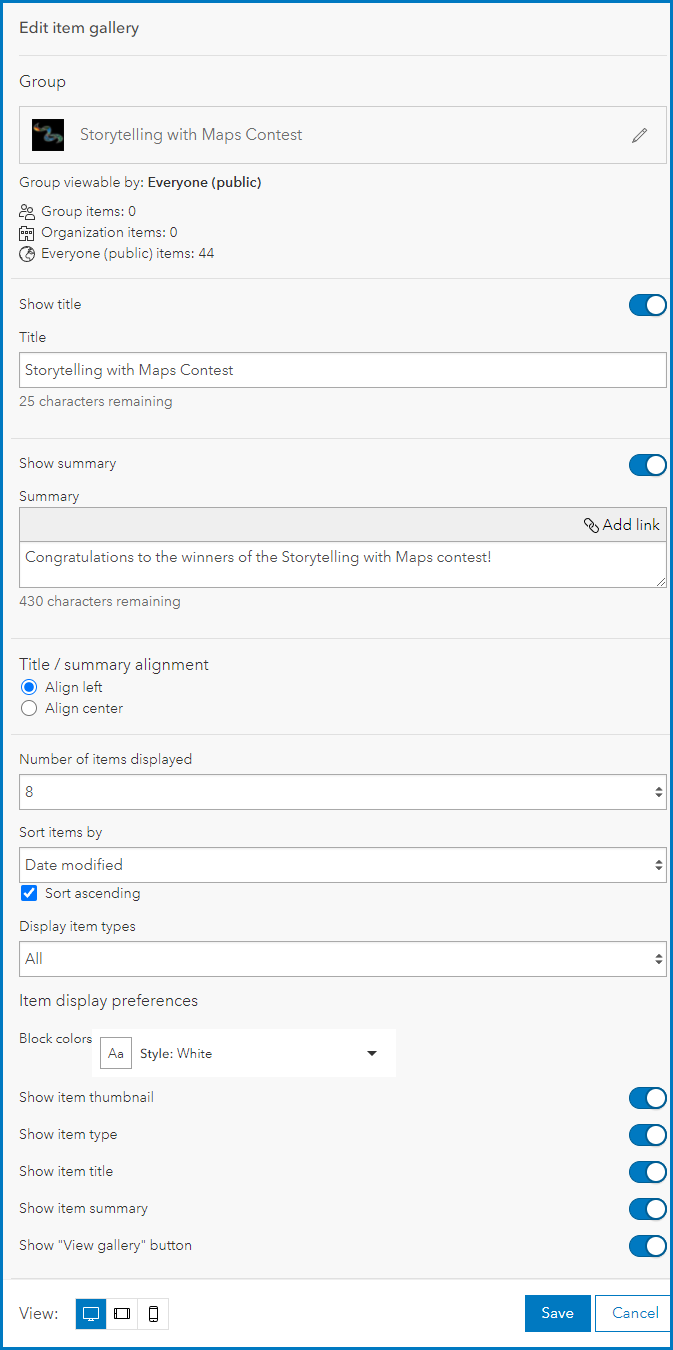The image is a detailed vertical screenshot of a user interface for an "Edit Item Gallery" feature. The screenshot displays a box with a very thin blue border around it, and at the top left-hand corner, it says "Edit Item Gallery." Below this heading, there's a section labeled "Group," which includes a small black box with a blue squiggle and the text "Storytelling with Maps Contest" to its right. The group is noted to be public, indicated by the line "Group: Viewable by everyone (Public)."

The information within the group is divided as follows: Group items: 0, Organization items: 0, and Everyone (Public) items: 44. The "Show Title" toggle is set to "on," and a summary section reads: "Congratulations to the winners of the Storytelling with Maps Contest."

In the top right corner, there is an option to "Add a Link," accompanied by a link icon. The interface indicates there are 430 characters remaining for further description or content.

Next, the section titled "Title/Summary Alignment" offers two options: "Align Left" in blue and "Align Center." Currently, eight items are displayed under "Number of Items Displayed." Users can sort these items by various criteria, although the default selection is "Date Modified" from a drop-down menu, with a checked blue box for "Sort Ascending."

Further down, the interface presents an option to "Display Item Types," defaulting to "All" as selected from a drop-down menu. Under "Item Display Preferences," the block color is set to white, and several display options are checked and slid to the right. These include: "Show Item Thumbnail," "Show Item Type," "Show Item Title," "Show Item Summary," and "Show View Gallery Button."